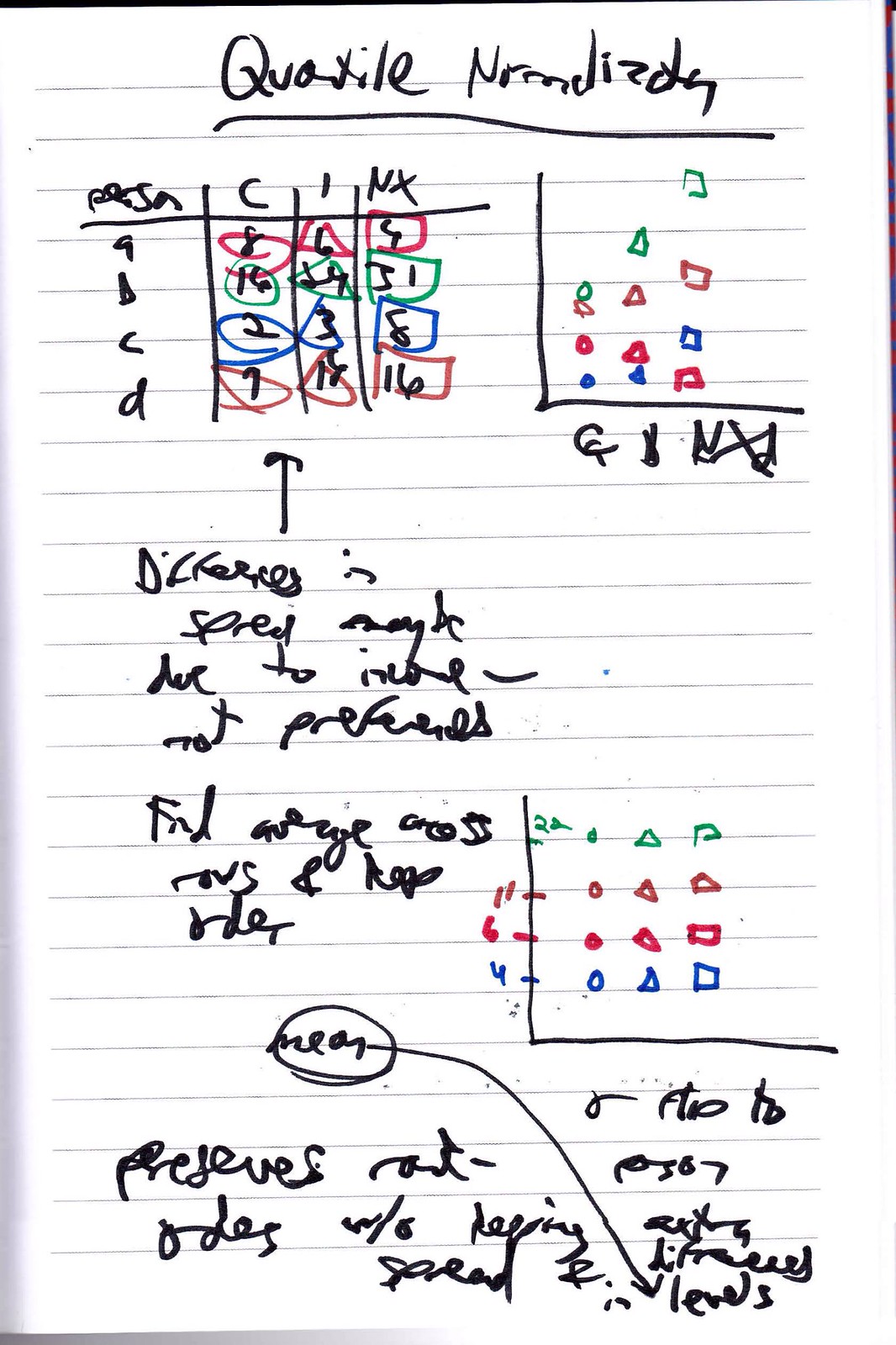**Detailed Caption:**

The image features a piece of white, lined paper with black horizontal lines. At the top of the paper is a title, underlined with a horizontal line drawn neatly beneath it. Below the title, there is a table filled with numbers, which are circled in various colors including red, green, blue, and brown markers. To the side of this table, there appears to be another table or possibly a graph, similarly marked with red, green, blue, and brown markers. Below these sections, more text is written in black marker, leading to another graph, followed by additional illegible text. The handwriting throughout the paper is difficult to read, but the use of different colored markers highlights specific elements within the tables and graphs.